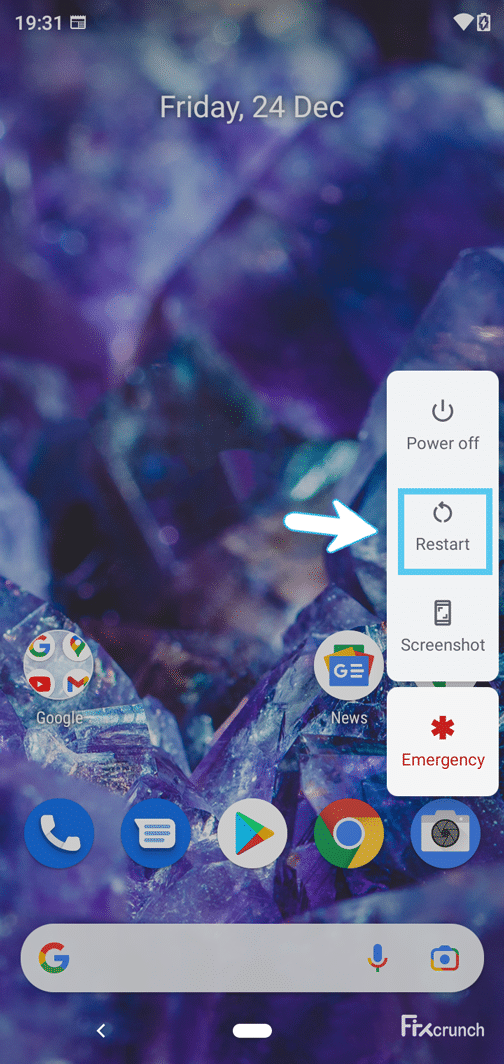Caption:

This is a screenshot of a mobile phone's wallpaper. The time is displayed on the upper left corner as "19:31" in white font. Adjacent to the time, slightly towards the right, there is a small square icon. On the upper right, the status bar icons for battery and Wi-Fi are clearly visible.

Centered at the top of the screen, with approximately four spaces before it, the date is shown as "Friday, 24 Dec" in white font. Both the "F" in "Friday" and the "D" in "Dec" are capitalized.

On the left side of the screenshot, there is a vertical options bar. This bar contains four distinct options: "Power off" at the top, immediately followed by "Restart", then "Screenshot", all listed vertically. Below these options, separated by a slight gap, there is a single item labeled "Emergency."